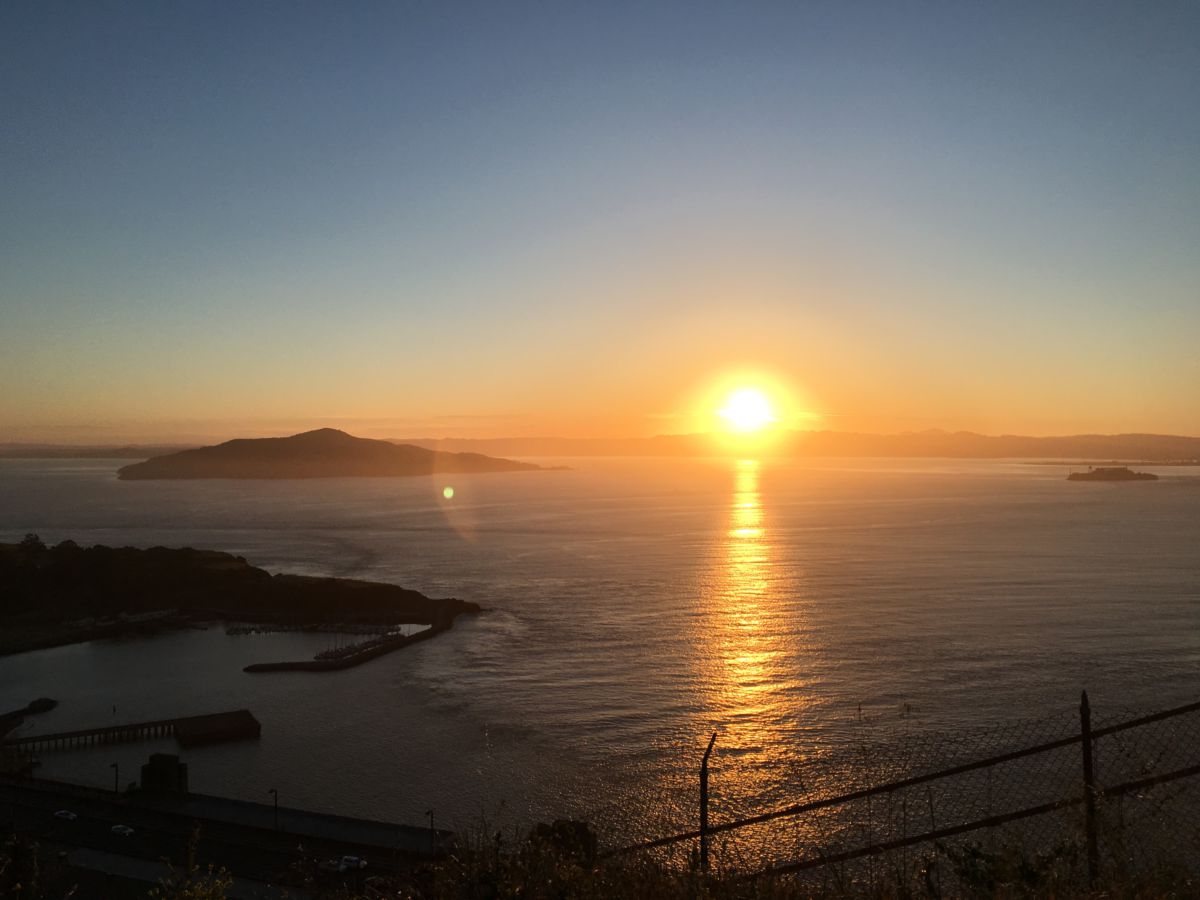This photograph captures a serene and picturesque scene at either sunrise or sunset, with the sun positioned very low on the horizon, casting an enchanting glow across the landscape. The sky is a gradient of colors, transitioning from a clear, dark blue at the top to a warm orange hue near the horizon. The sun itself shines brightly, with a nearly white center surrounded by vibrant yellow tones. Below the horizon, the calm, almost flat surface of a large body of water reflects the sunlight, adding to the tranquility of the scene. Slight ripples gently break the water's surface. 

Prominently featured in the scene are rocky islands, one large island jutting out to the left and a smaller one towards the center-right, adding depth to the composition. In the foreground, the silhouette of a metal chain-link fence is visible on the bottom right, serving as a boundary for visitors near the cliff. Towards the bottom left, several wooden piers and harbors scatter along the bay, accompanied by boats nestled in the water, suggesting a maritime setting. The entire scene conveys a sense of peaceful isolation, accentuated by the absence of clouds and tall buildings on the distant islands, resulting in a beautifully clear and unobstructed view.